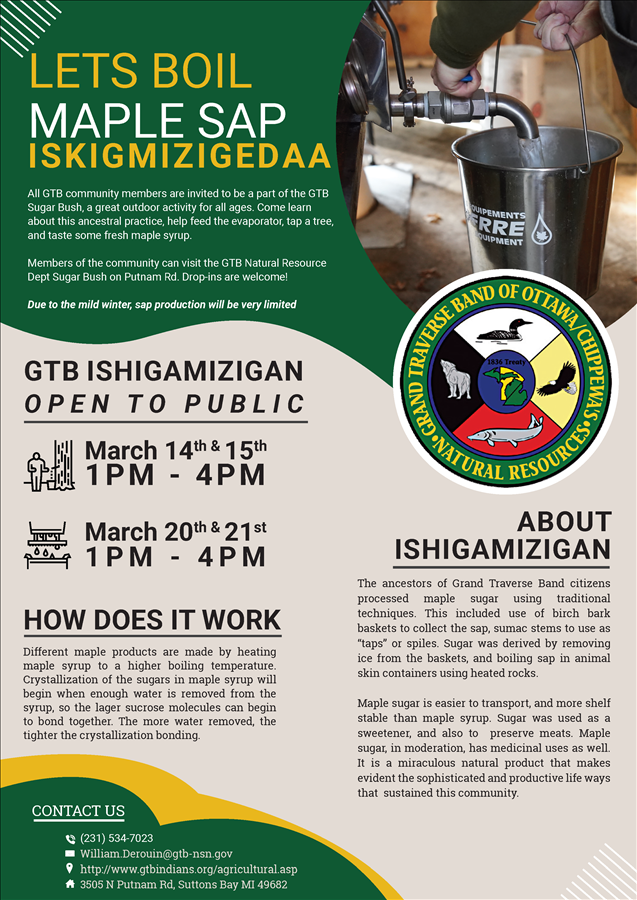This detailed advertisement flyer for a maple sap boiling demonstration features a serene and rustic theme predominantly colored in rich greens, tan, and cream with touches of yellow. The headline at the top reads, "Let's Boil Maple Sap," with "eskigmizigeta" highlighted below it. In the upper right-hand corner, there's a vivid image of a silver tap inserted into a tree, with a clear liquid pouring into a silver bucket held by someone’s hands. This scene is set in an old wooden room filled with various buckets and equipment, adding to the rustic charm. The flyer includes an insignia of the Grand Traverse Band of Ottawa Chippewa's Natural Resources, depicting a wolf, a duck, an eagle, and a sturgeon. Important dates for the public demonstration are clearly listed: March 14th and 15th as well as March 20th and 21st, from 1 p.m. to 4 p.m. A section titled "How Does It Work?" provides a detailed explanation of the sap boiling process, and contact information is available in the bottom left corner. The top portion of the flyer has a red overlay which aids in drawing attention to the event.